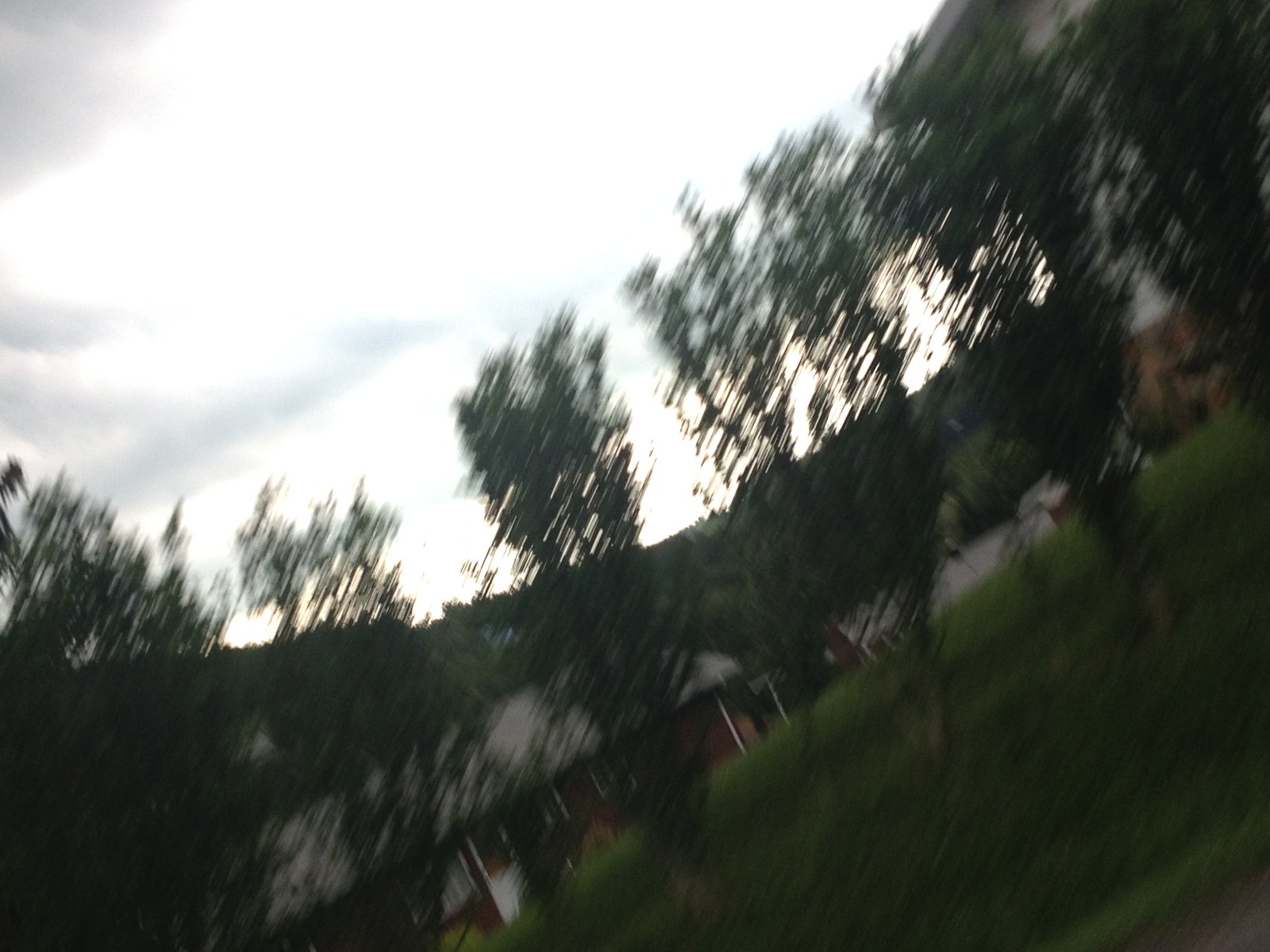This photograph, though quite blurry, depicts a rustic outdoor scene. In the foreground, a row of trees, reminiscent of those used as natural property dividers, can be seen. These trees, while not distinctly visible due to the blur, suggest a sense of separation and privacy between adjoining lands. Behind this line of trees, a brown rambler house is noticeable, partially occluded by the foliage. The sky above is overcast with grayish clouds, adding a somber tone to the setting. Interestingly, the photo is tilted at a 45-degree angle, giving an unconventional perspective to the viewer. On the right side of the image, another rambler-like structure appears, hinting at a possible farmhouse setting. This secondary building reinforces the rural ambiance of the scene. Despite the lack of text, the image vividly portrays a serene yet slightly disoriented snapshot of country living.